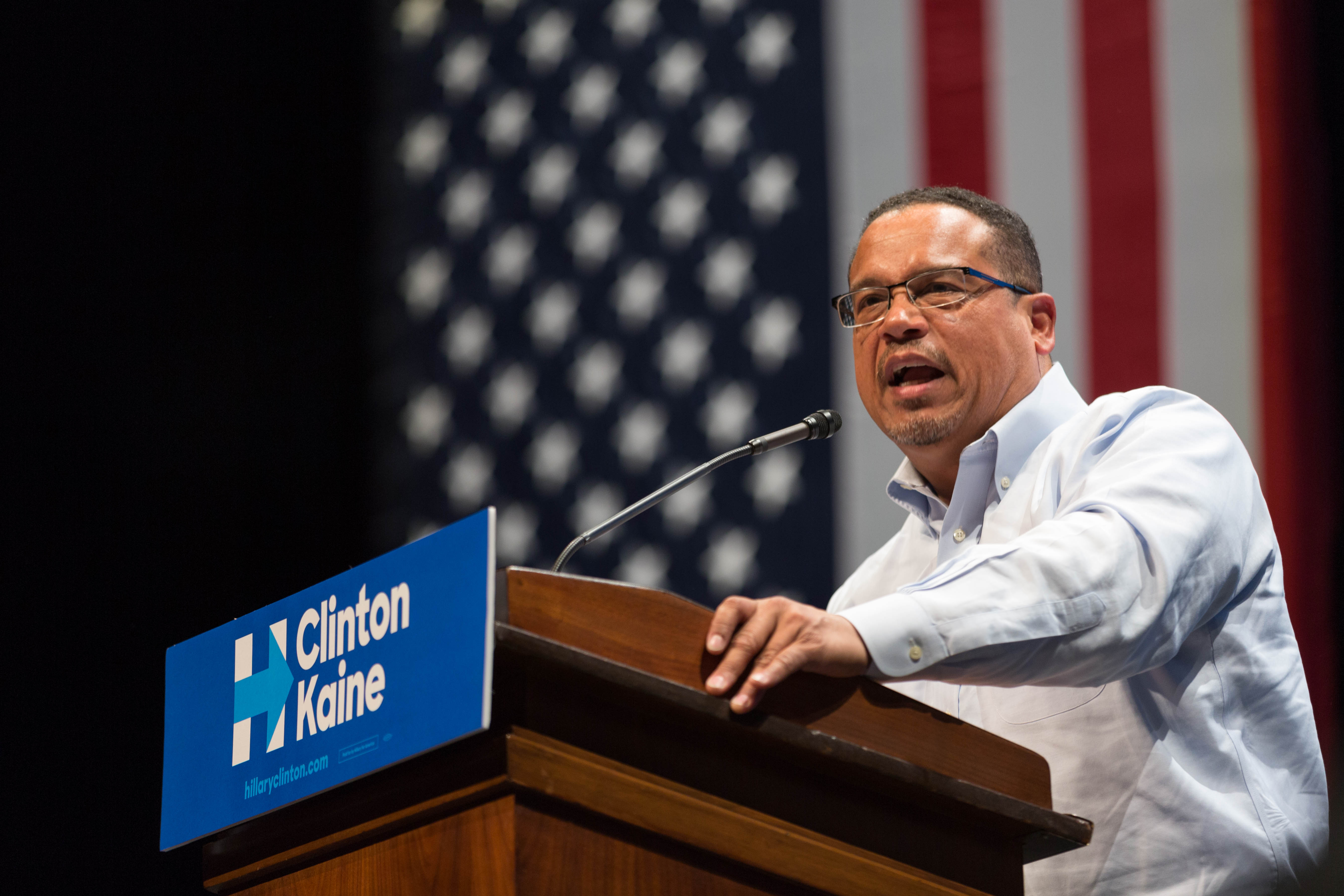The image captures a male with tanned skin and short black hair, wearing glasses, standing behind a wooden podium with a rich brown hue. Centered on the front of the podium is a blue banner that reads "Clinton Kane" in bold white letters. To the left of the text is a white "H" logo with a blue arrow shooting through it, captioned with "hillaryclinton.com." The man is dressed in a light blue shirt with the top button undone. He stands with his left hand resting on the podium, his mouth open as if addressing an audience through the microphone positioned in front of him. The background is stark black, accented by an American flag with its iconic red and white stripes and a blue rectangle filled with white stars suspended behind him.